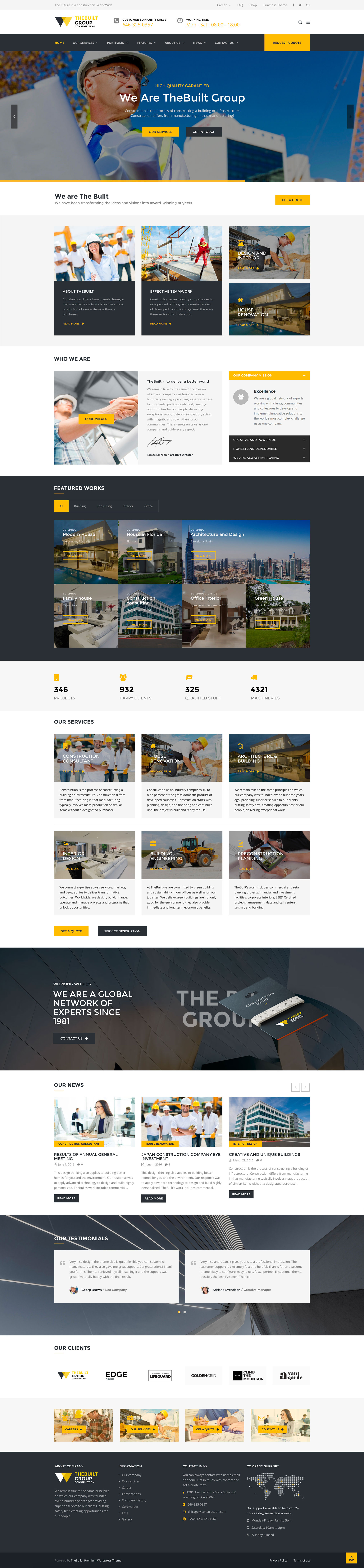The image showcases a web page belonging to a business called 'The Built Group,' located at the top left corner along with their logo. The main heading reads, "We are The Built Group." A prominent feature of the page is a man wearing a construction hat and glasses, dressed in a white shirt and blue tie. Surrounding him, the text highlights impressive company statistics, including "346 projects," "932 happy clients," "325 qualified staff," and "4,321 machineries." The color scheme prominently features shades of yellow, black, white, and blue. In the background, there are images of buildings and construction sites, visually representing the company's industry and capabilities.